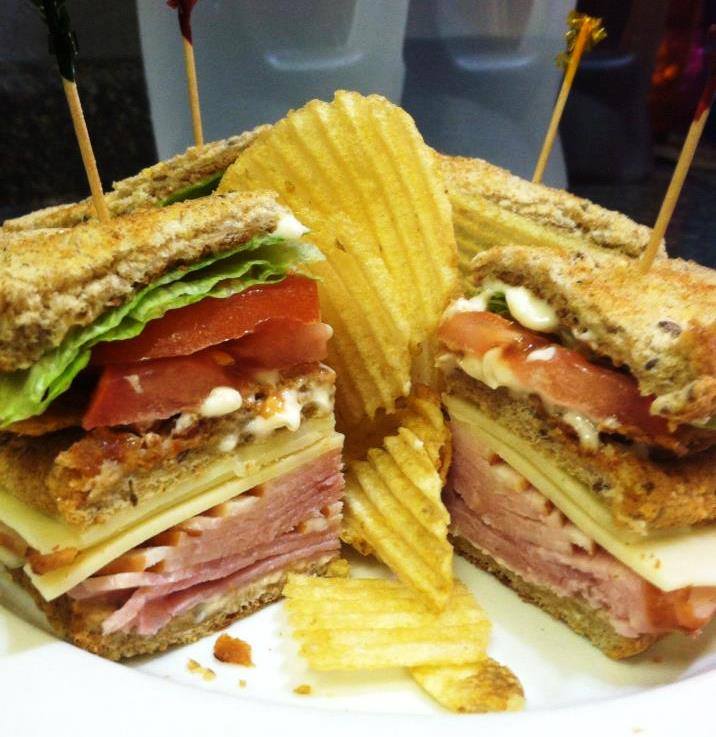This is a close-up photo of a club sandwich cut into quarters on a white plate. Each quarter is secured with a toothpick, with two being black, one yellow, and one red. The sandwich features toasted, golden brown whole wheat bread, layers of a pinkish ham, white cheese slices, green lettuce, red tomato, and a dollop of white mayonnaise. Golden, ridged potato chips are scattered around the sandwich pieces on the plate. The background is predominantly dark on the right and left, with a white object in the center. Behind the plate, two blue plastic cups can be seen, adding a hint of color to the dark backdrop.